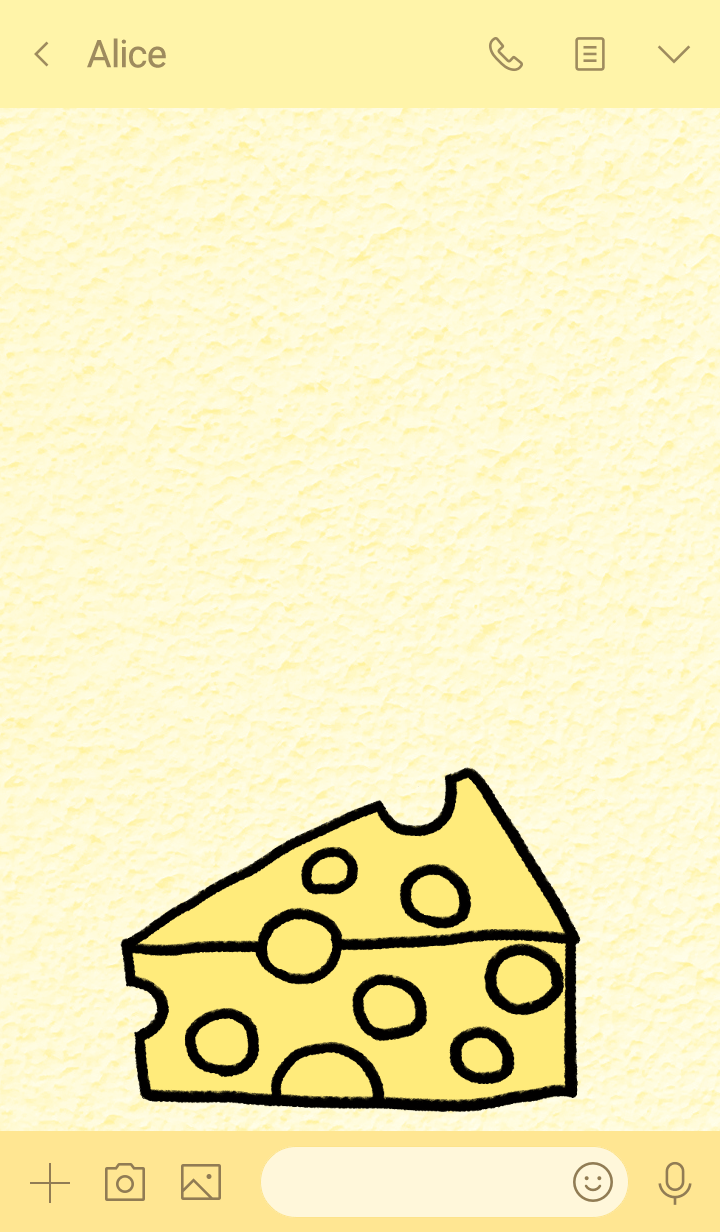The image appears to be a screenshot from a chat application on a mobile device, likely Android, displaying a pale yellow background with a distinctive textured pattern resembling a popcorn wall. The screen is structured with a header at the top, reading "Alice" in a darker yellow bar. To the right of "Alice" are three icons: a phone symbol, an outline of a document, and a downward-facing arrow.

In the main section of the image, occupying about 80% of the screen, there is an illustration of a slice of Swiss cheese, characterized by a darker yellow hue and black outline with holes. This illustration appears to be part of a conversation, potentially an image sent via the chat interface. The bottom of the screen features a darker yellow bar containing interactive icons including a plus sign, a camera, an image symbol, an oval-shaped input field for text, and a microphone icon, indicative of a messaging and multimedia application. The entire layout has a uniform yellow tint, adding to the visual coherence of the interface.